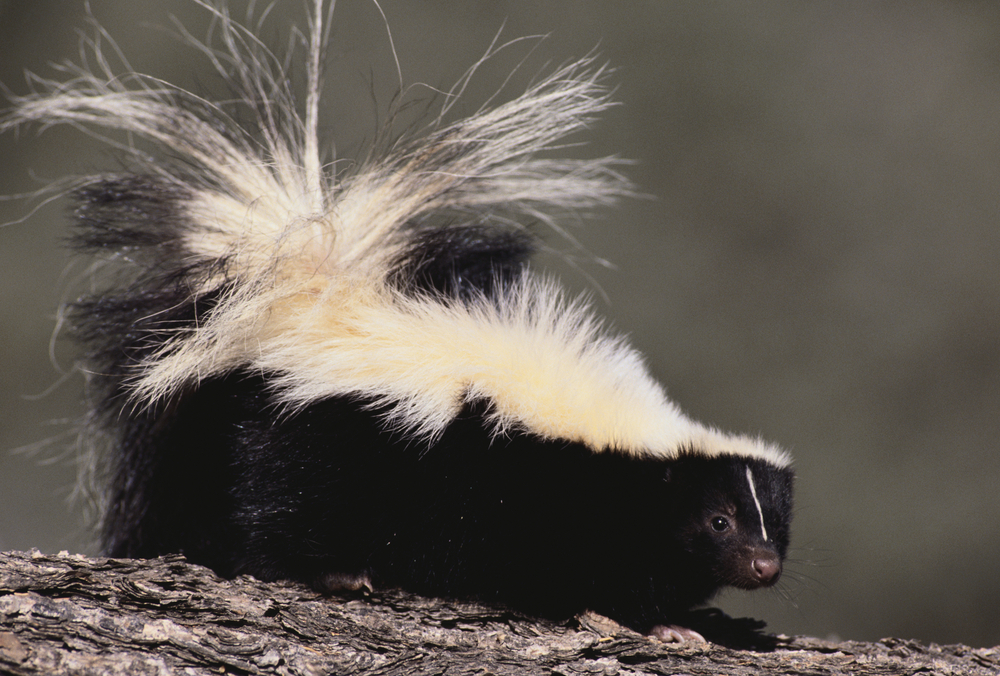In this detailed photograph, a skunk is captured walking low on a piece of textured tree bark. The skunk's fur is notably disheveled and frayed, adding to its rugged appearance. Its coat features a striking black and white pattern: the lower part of its body is predominantly black, while the top displays white fur interspersed with splotches of black. A solid white stripe runs from its forehead down to its lighter-colored nose. The skunk's eyes have dark pupils, and the area around its eyes is brown, matching its nose. Its gaze is directed towards the camera and slightly to the right. The tree bark underneath the skunk is light brown with splotches of tan, and its rough pattern is discernible both behind and in front of the skunk. The background of the photo is out of focus and dark, ensuring that the skunk remains the central focal point. The setting appears to be outdoors on a bright, sunny day, as indicated by the natural light highlighting the scene.